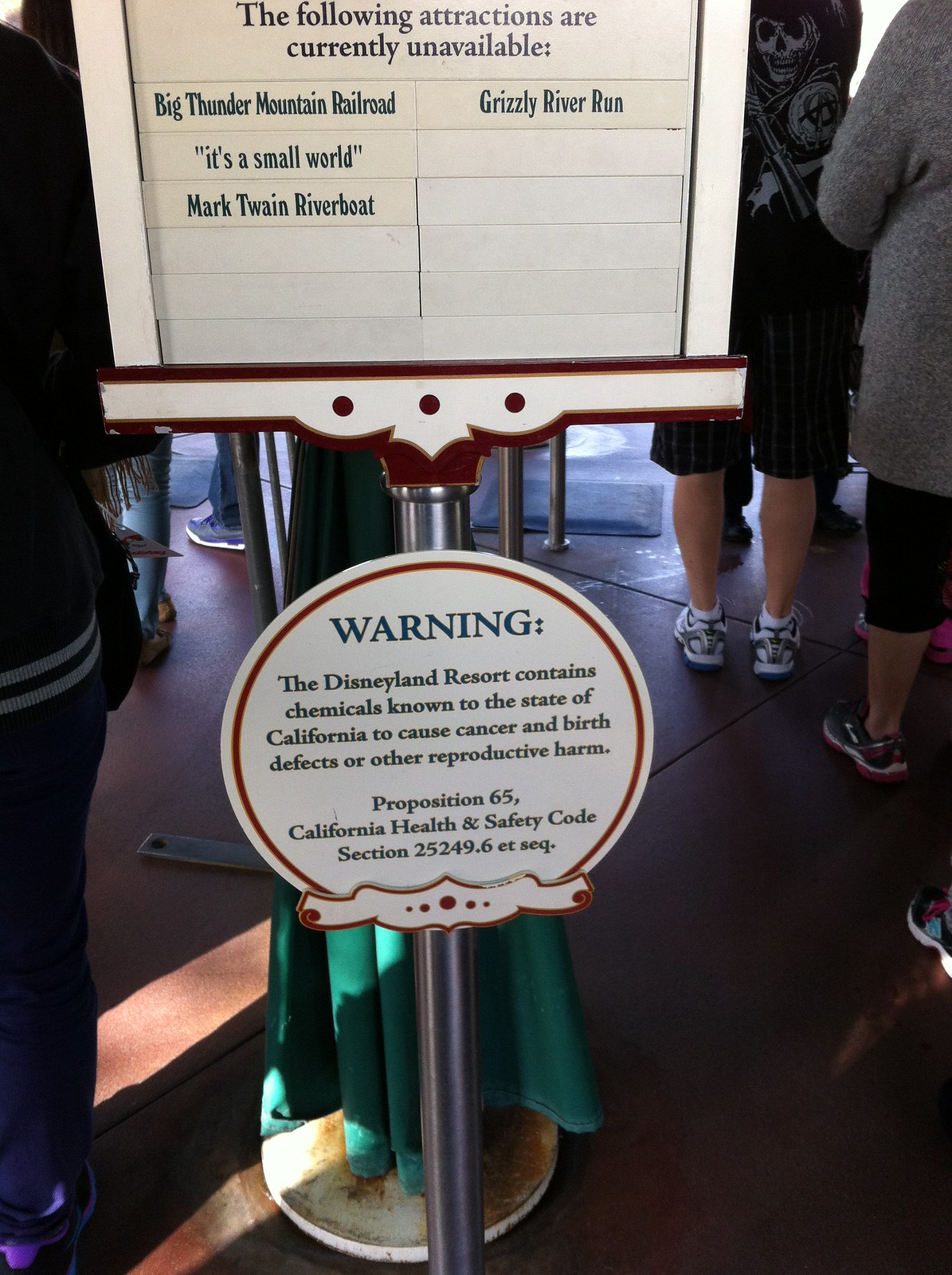The image depicts a bright, clear day at Disneyland, showcasing a prominent circular sign with a red border, primarily white in color. The sign announces that several attractions are currently unavailable: Big Thunder Mountain Railroad, It's a Small World, Mark Twain Riverboat, and Grizzly River Run. Beneath this list, a warning is displayed, informing visitors that the Disneyland Resort contains chemicals known to the State of California to cause cancer, birth defects, or other reproductive harm, in accordance with Proposition 65, California Health and Safety Code Section 25249.6 ETSEQ. The scene also includes partial views of several people, including a boy and a woman, captured from the shoulders down, standing as if they are waiting in line, adding a sense of anticipation to the overall atmosphere of the well-lit setting.